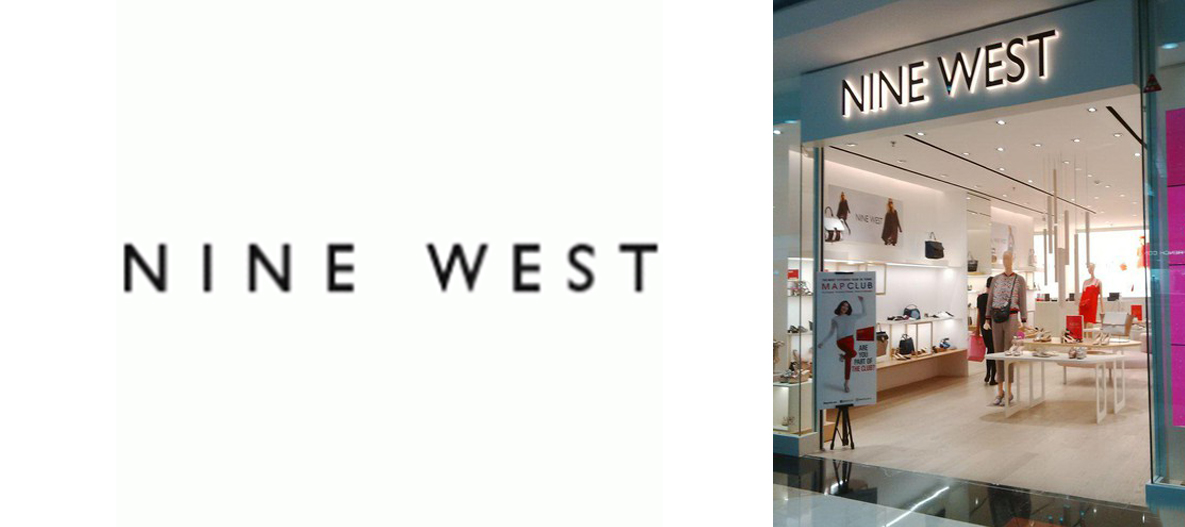The image features a storefront for Nine West, prominently located inside a mall. On the left side of the photo, there's a plain white background with the brand name "Nine West" in black, evenly spaced, all-capital letters. To the right, a well-lit, predominantly white Nine West store interior can be seen through its entrance. The store's name is also displayed in black capital letters, illuminated from behind, above the entrance.

Inside the store, mannequins dressed in various outfits are positioned near the front, alongside tables displaying shoes and handbags. The store’s layout includes white walls and ceiling, accented by vibrant spotlights. At the entrance, there's a poster featuring a woman in red pants and a white shirt kicking her leg up behind her, alongside the text "Map Club." Additional signage and displays are visible, including a pink banner in the store window and a taupe-clad mannequin near the front. In the background, closer to the counter, another mannequin wears a red outfit. A red display adds a pop of color amid the overall white decor, while the cash register area is located at the back of the store. The floor transitions from the black of the mall to the white interior of the store, further delineating the space.